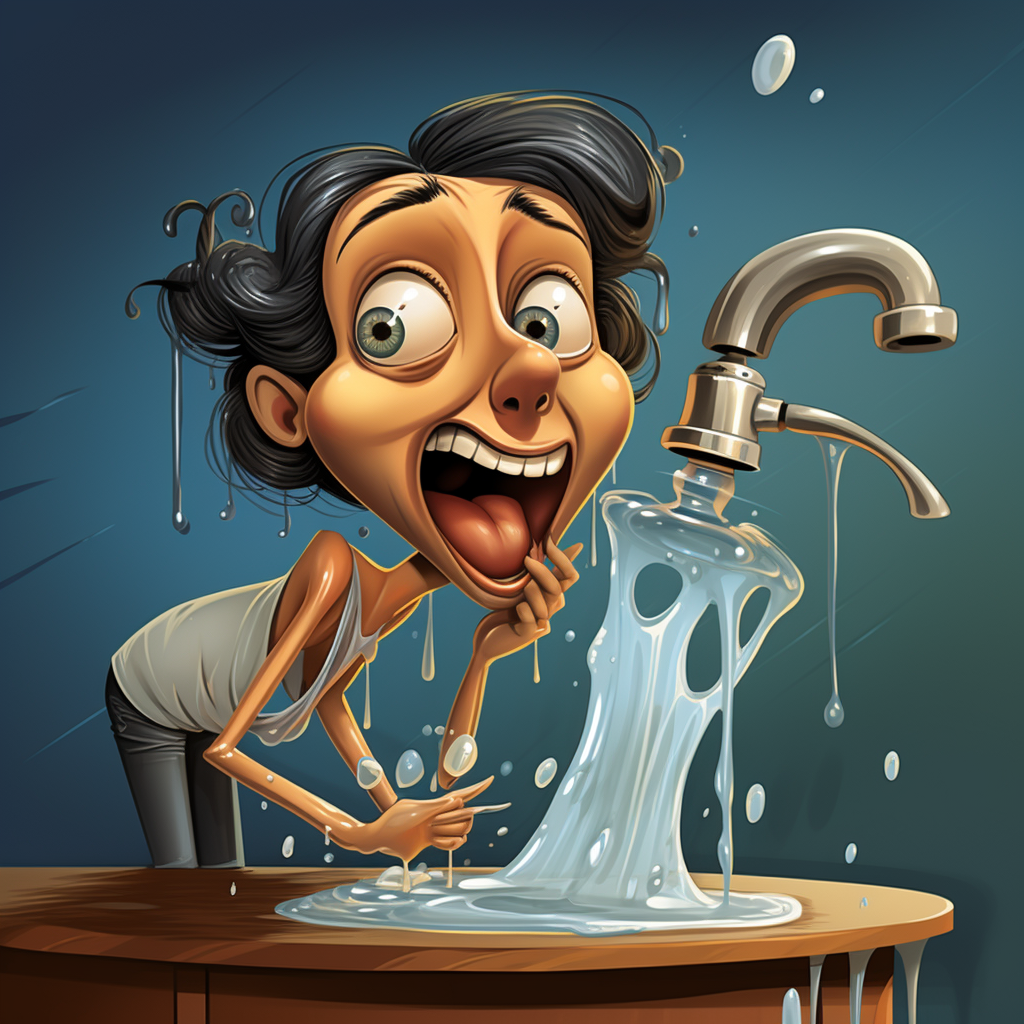This is a detailed cartoon drawing set against a dark grayish blue background, lighter in the middle. It features a woman with a surreal and alarming expression. Her eyes are bulging out, wide open, and looking to the left. Her mouth is agape, visibly showing her teeth and tongue, as if she's yelping in shock or calling for help. Her left hand is raised to her mouth, fingers splayed in alarm. She has short, dark gray hair, and blue eyes, which contrast sharply with the background.

The woman, who appears to be a modern housewife, is wearing a light gray tank top and dark gray pants. Her arms are skinny, and her head appears unusually large compared to her thin body. 

In front of her, a silver faucet is floating mid-air, detached from any sink, with a torrent of water gushing out unchecked. The liquid cascades over a table and splashes everywhere, adding to the chaotic scene. Water droplets are even dripping from her hair, emphasizing the extent of the mess. The overall imagery conveys a sense of horror and surrealism.